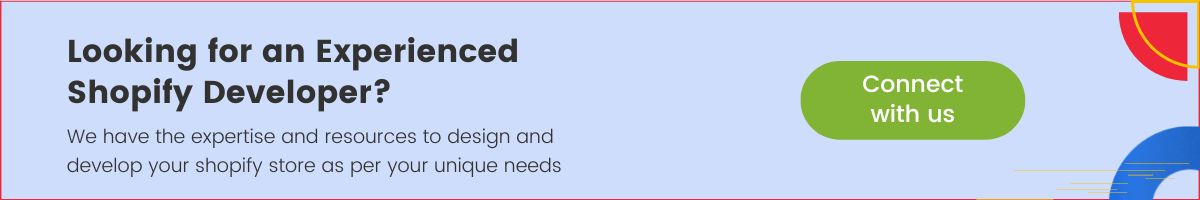A light blue ad box, bordered by a red line, prominently features black text that reads, "Looking for an experienced Spotify developer?" in bold, larger font at the top. Below, a smaller, subtle font explains, "We have the expertise and resources to design and develop your Spotify store as per your unique needs." Towards the bottom right of the ad, a green button with white text invites viewers to "Connect with us." In the corners, a red spot and a blue spot add additional visual elements.